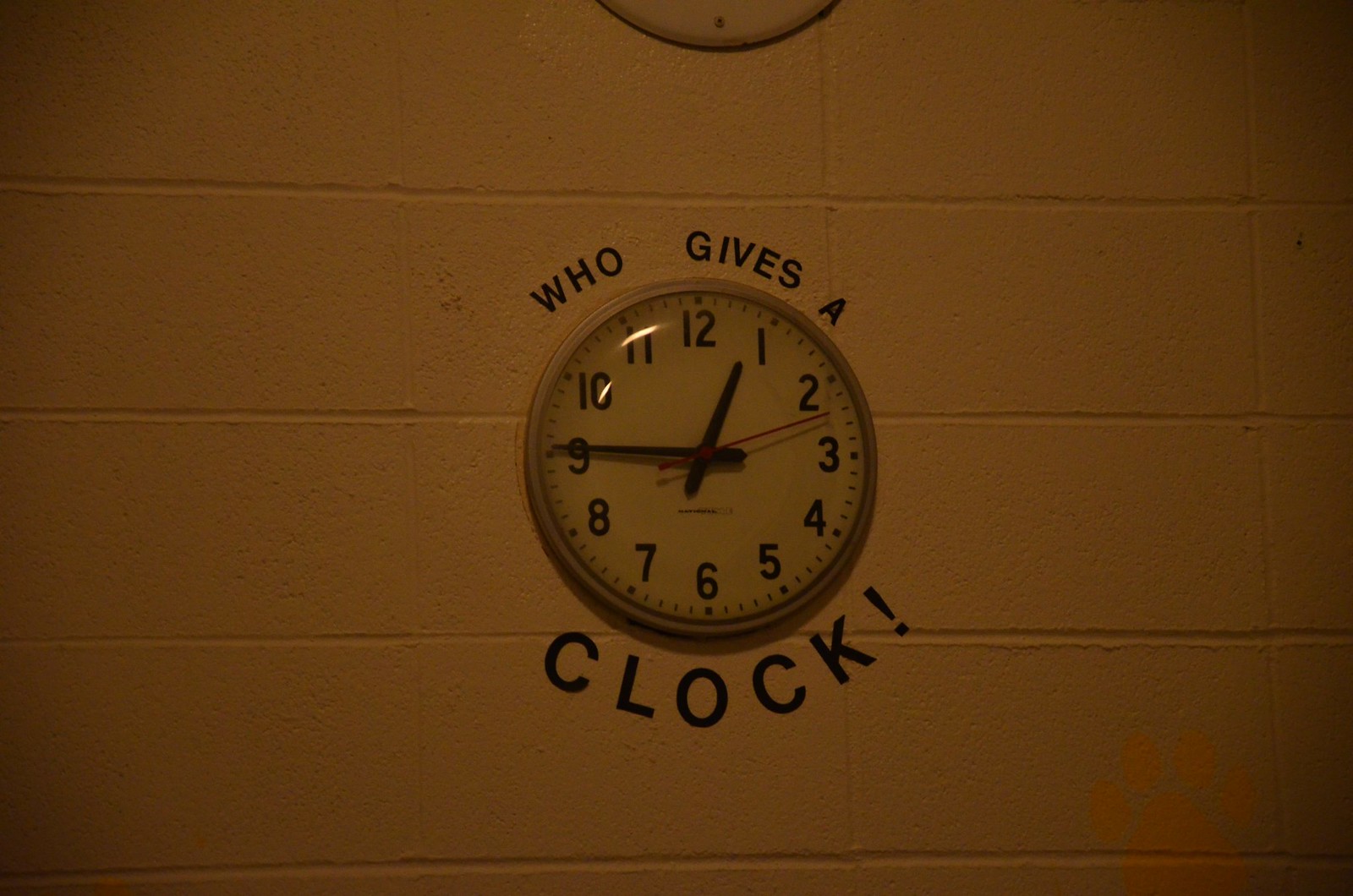A detailed photograph features a classic circular clock mounted on a white brick wall, reminiscent of those commonly found in high school settings. The clock has a white face with black numerals from 1 to 12, black hour and minute hands, and a distinctive red second hand. The time displayed is approximately 1:45 to 1:46. Encircling the numerals, in a mix of smaller and larger letters, the clock bears the quirky phrase "Who gives a clock!" with an exclamation point emphasizing the punchline. Above the clock, another circular object is partially visible at the very top of the image, though only its bottom edge can be discerned, leaving its identity ambiguous.